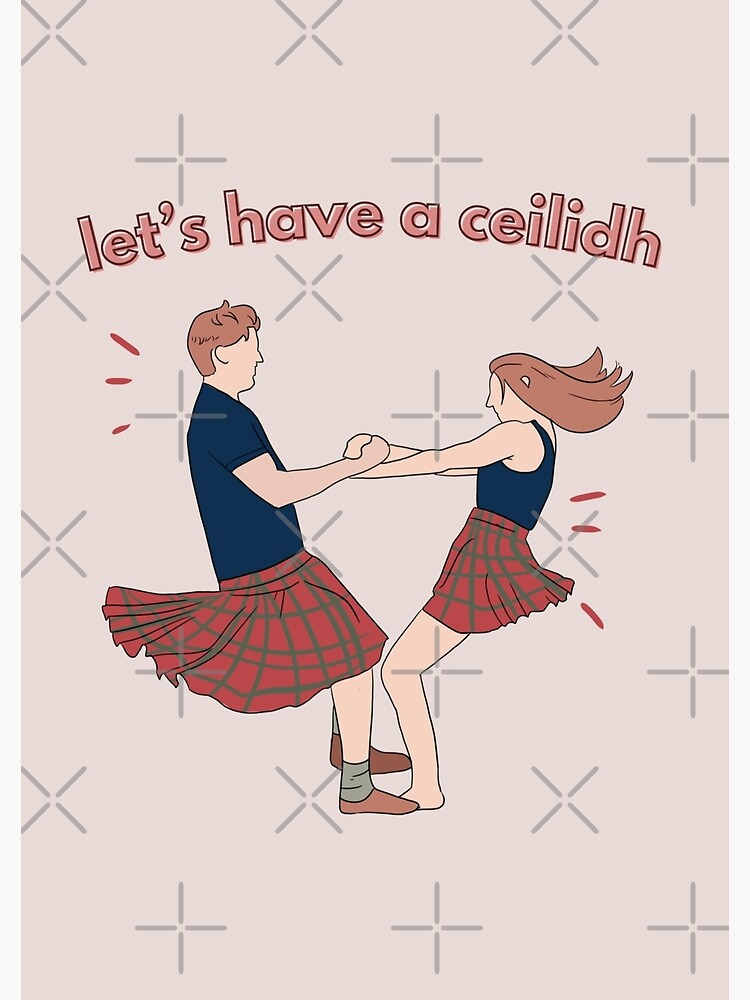This image, likely an invitation, is a vertically-oriented rectangle measuring approximately 6 inches high by 4 inches wide, with thin light gray borders flanking each side. The background is a pale mauve, blending pinkish tones with a gray undertone, and patterned with subtle gray X's and plus signs serving as a faint watermark.

At the top of the image, stylized red lettering with a white outline arches gracefully, reading "Let's have a CÈILIDH," a Gaelic word for a social gathering or party. Below this, a charming illustration depicts a man and a woman engaged in a lively dance. Both figures have brown hair; the man sports a short-sleeved blue shirt and the woman wears a blue tank top. Each of them is clad in traditional red plaid kilts with dark green lines, symbolizing their cultural heritage. They are linked arm-in-arm, swaying in a manner suggesting a joyful swing dance. Despite the lack of detailed facial features, their locked arms and animated poses convey a sense of exuberance and movement, enhanced by motion lines in the background. The image as a whole exudes a festive, inviting atmosphere, characteristic of a traditional Scottish or Irish celebration.